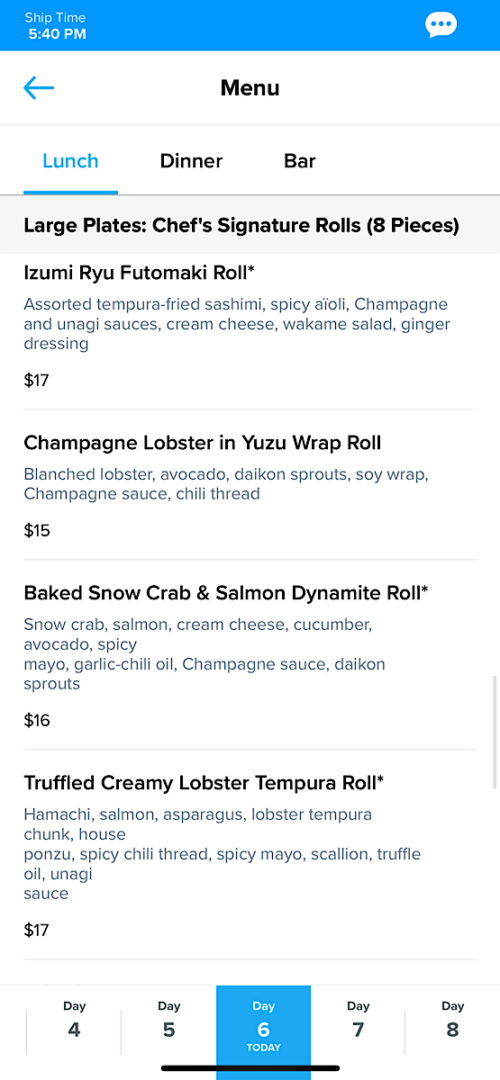Screenshot of a dining app or website displayed on a smartphone at 9:40 PM. In the top left corner, the phone's time is visible alongside standard interface elements like signal bars and battery percentage. At the top right, there is a notification symbol featuring three dots and a speech bubble.

The focal point of the image is the menu section of a restaurant, indicated by a large header that reads "Menu." Below this header, the menu is segmented into three distinct tabs: Lunch (highlighted in blue), Dinner, and Bar, suggesting organized meal options depending on the time of day or dining preference.

In the highlighted Lunch tab, specific items are listed under the category "Large Plates" and "Chef's Signature Rolls (8 pieces)." Four sushi rolls are prominently displayed:

1. Izumi Ryu Futamaki Roll - $17
2. Champagne Lobster and Yuzu Wrap Roll - $15
3. Baked Snow Crab and Salmon Diamond Roll - $16
4. Truffled Creamy Lobster Tempura Roll - $17

The exotic names and relatively high prices of the dishes imply that this is likely a Japanese or possibly a fusion Asian restaurant, offering a gourmet dining experience.